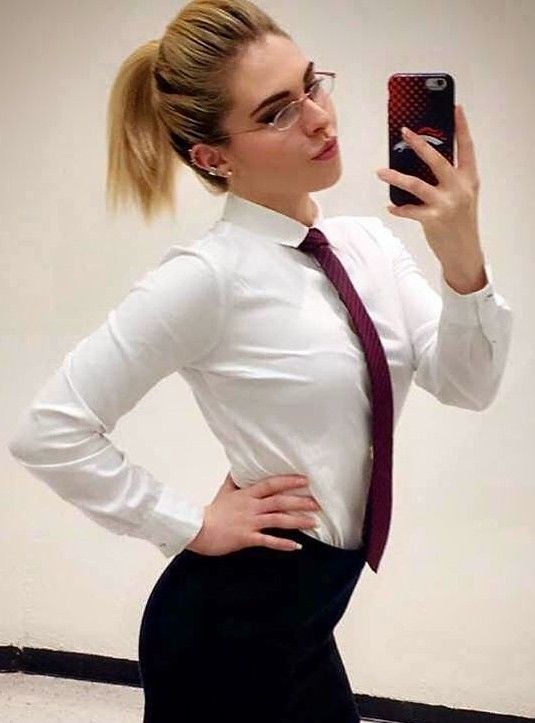In this vertically-oriented photo, a woman in her twenties is confidently posing for a selfie, holding up a smartphone with a distinctive Broncos case in her left hand close to her face. She has dirty blonde hair, featuring black roots, styled into a poofy ponytail. Her attire is business-like: she's wearing clear-rimmed, thin white glasses and has multiple earrings visible in her ears. She sports a tight white collared button-down shirt that extends to her wrists, paired with a maroon tie. Her high-waisted black pants emphasize her posture as she places her right hand on her hip. The backdrop features an off-white wall with a black border at the bottom. The floor beneath her, though not fully visible, appears to have off-white and grayish designs. She exudes confidence, accentuated by her lightly made-up face and the subtle "duck face" expression she's making.